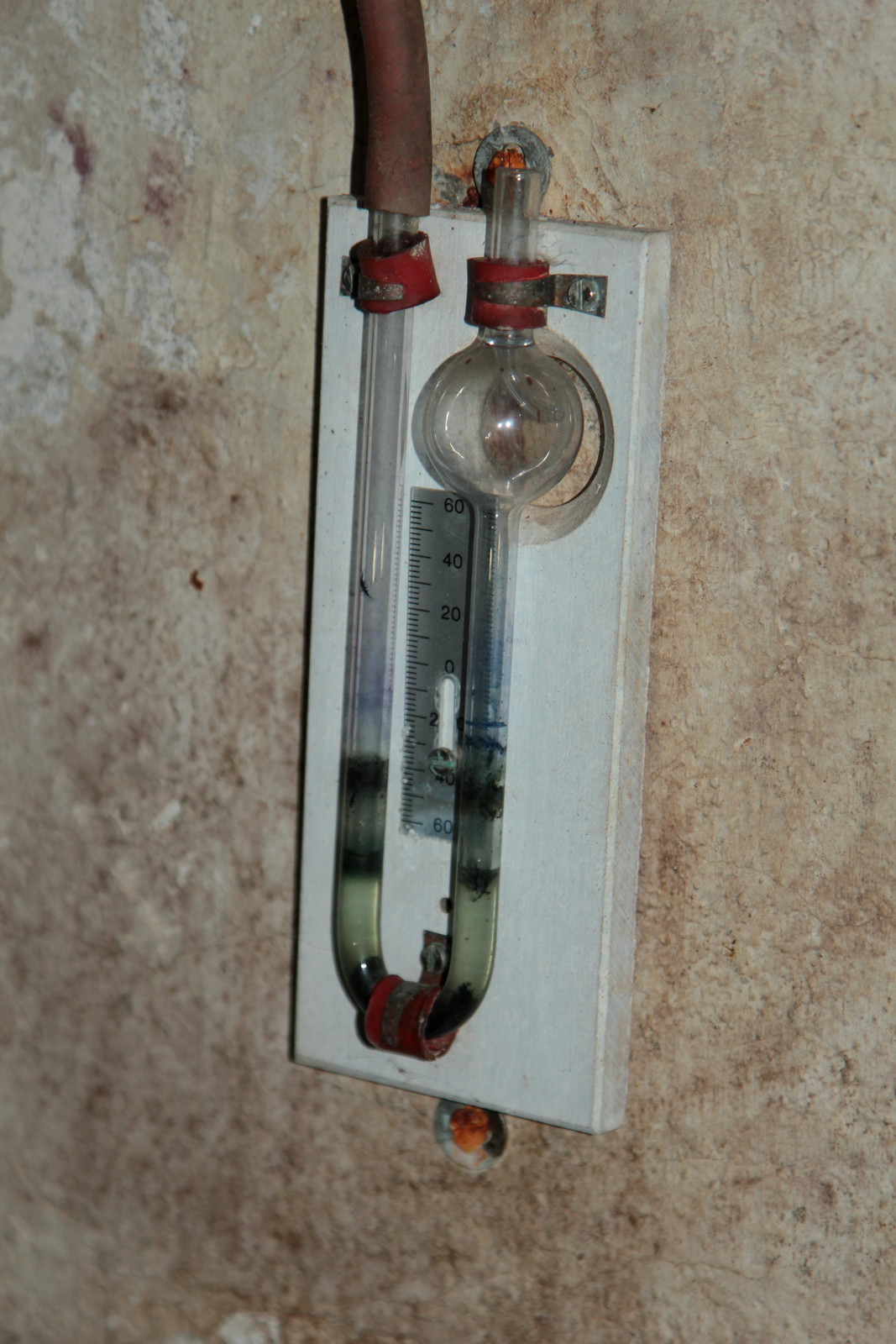The image depicts a square white plastic box positioned against a background that appears to be either cement or granite, making it unclear whether the box is mounted on a wall or placed on a floor. The box contains a measurement gauge designed to track gases or fluids. 

On the top left edge of the box, there's a brownish rubber stopper attached to the end of a transparent tube, made of either glass or plastic. This tube descends along the left side of the box, curves at the bottom to form a U-shape, and then rises back up through the center of the box. The tubing ends in a circular clear glass component that houses a silver ball. 

Just above this circular area, two red bands encircle the tubing. They rise slightly above the top of the box before curving to the rear. Nestled in the crook of the U-shaped tubing is a small silver rectangular element, which features measurement lines on its left side. The right side of this silver piece displays black numerical markings: 0, 20, 40, and 60.